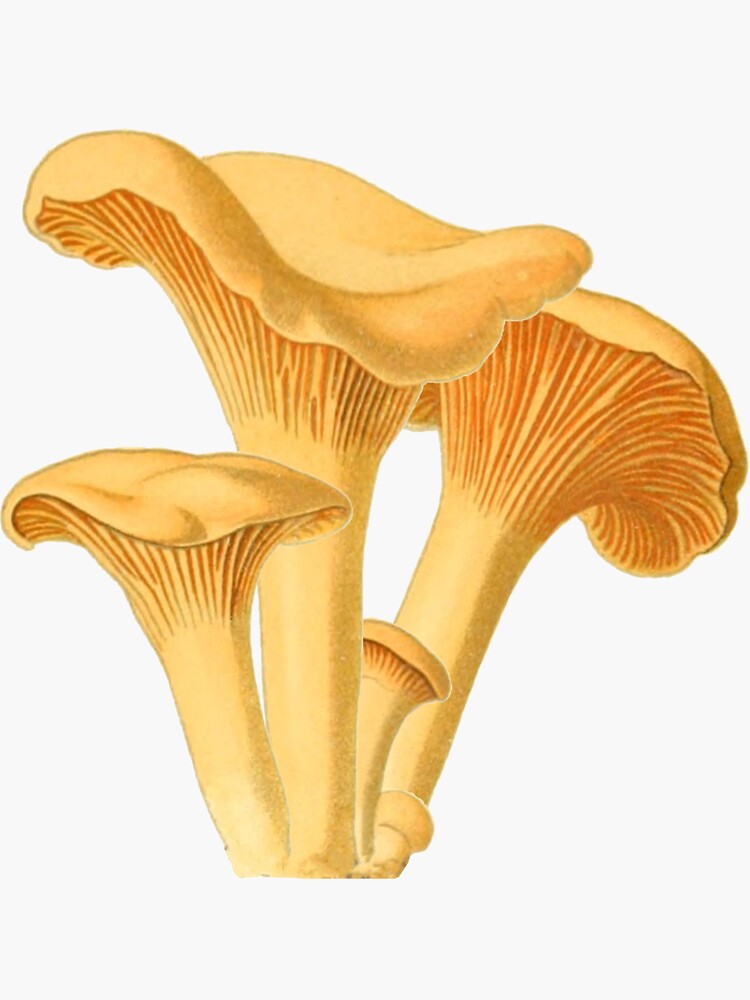This image is a detailed vertical rectangle illustration with a nearly white background, slightly leaning towards very light beige or gray. Dominating the scene are five hand-drawn, yellowish-beige mushrooms with wavy tops, arranged in a clustered manner. They vary in size: there are two tall mushrooms with one central and another on the right, a medium mushroom midway up between the tallest ones, a smaller mushroom to the left coming just below the central tall mushroom, and a tiny one nestled at the base. The mushrooms exhibit intricate details, with their stems smoothly transitioning into furrowed ridges as they ascend toward the caps, which drape gracefully over the top. The ridge lines beneath the caps are more of a reddish hue. The overall color palette of the mushrooms ranges from light to dark brown, with the deepest browns highlighting the furrows and shadows. The artwork lacks any background elements or text, emphasizing the elegantly fluted mushrooms in a clean, minimalist setting that accentuates their hand-painted, animated style.